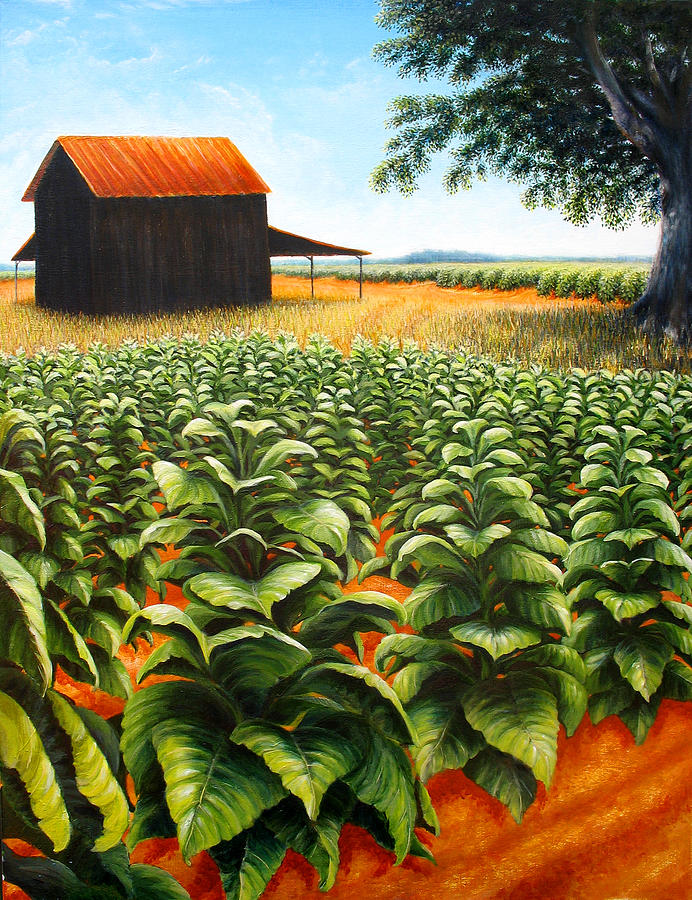This vertical rectangular artist's conception vividly portrays a serene, rustic farmland scene. In the foreground, rows of waist-high plants with large, lush leaves stretch out, their greenery contrasting against the brownish-orange soil. These plants, possibly crops, have been meticulously plowed and planted, reflecting a well-tended agricultural field.

Beyond this cultivated land, wild natural grass encircles the field, adding a touch of untamed beauty to the scene. Dominating the top left of the painting is an old wooden barn with dark hued sides and a corrugated tin roof, which has weathered into shades of rusty orange and yellow. The barn features overhangs on both sides, providing much-needed shade.

In the distance, another expansive field mirrors the foreground crops, extending as far as the eye can see, suggesting vast farmland. To the upper right of the painting stands a tall, majestic oak tree, its leaves sprouting at the branch ends, adding to the overall impression of a lush, vibrant spring or summertime setting. The land is flat, extending uninterrupted to the horizon under a bright blue sky, encapsulating the serene beauty and diligent cultivation of rural life.